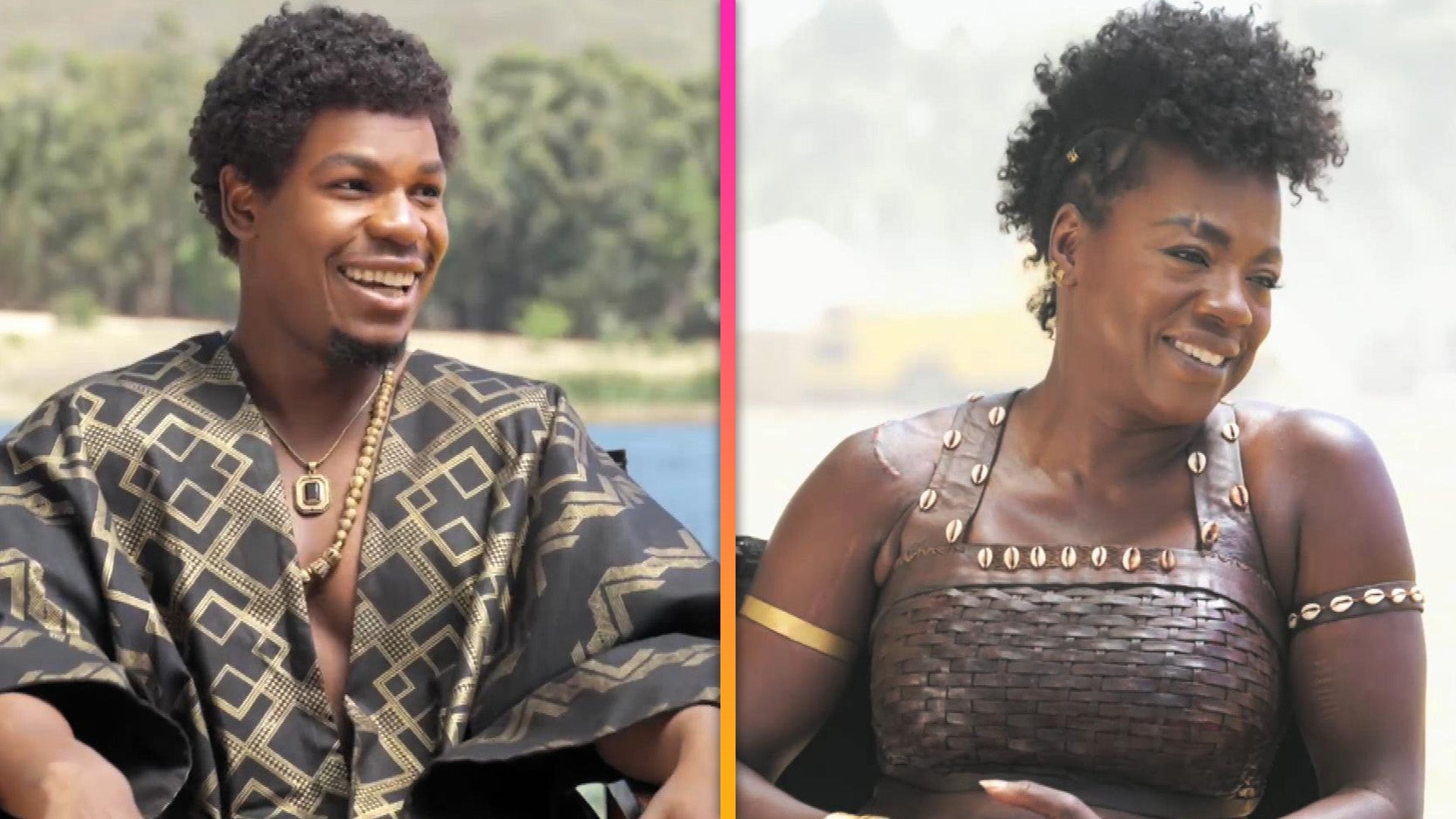This diptych image features two people of African descent, each positioned on either side of a thin vertical stripe that transitions from bright pink to orange and finally gold. 

On the left side, there's a waist-up photograph of a man with a broad smile, facing slightly to the right. He has short, curly black hair and a goatee. He is wearing a black and gold loose-fitting robe adorned with gold geometric patterns and an assortment of gold jewelry, including a beaded necklace and a pendant. Behind him, the background is an outdoor daytime setting, showcasing a serene lake with clear water and a line of green trees.

On the right side is a woman seen from the mid-torso up. She has her black curly hair styled in a mohawk fashion, with the sides braided close to her scalp. She is smiling and looking down towards the lower right. She is dressed in a halter-style top with a basket weave print, embellished with what appear to be light brown shells or gold beads. Her upper arms are adorned with matching bracelets. The background behind her is whited out, giving a foggy and overexposed appearance.

Both subjects are depicted in traditional African clothing, adding cultural richness to the visual narrative.